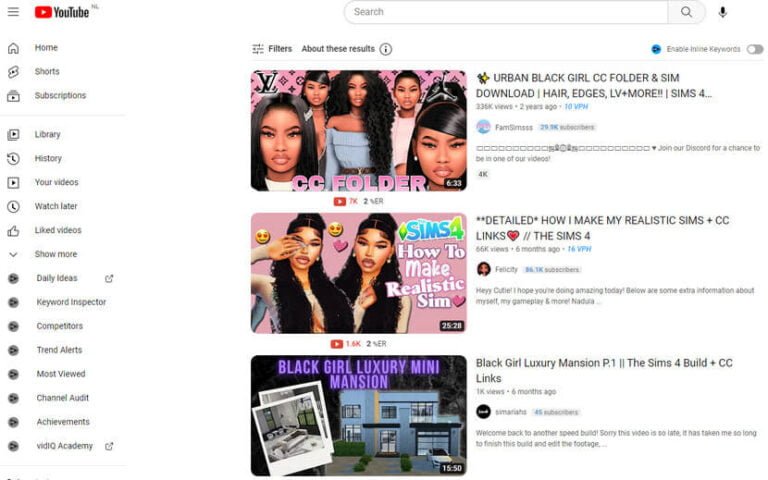This screenshot captures a YouTube page featuring a search bar at the top, which is currently empty. Three video results are prominently displayed. The first video is titled "Urban Black Girl CC Folder and Sim Download," the second is labeled "Detailed: How I Make My Realistic Sims," and the third video is "Black Girl Luxury Mansion: The Sims 4 Build." On the left side of the page, there is a vertical menu below the YouTube icon, listing various functions such as Home, Shorts, Subscriptions, Library, History, Your Videos, Watch Later, Liked Videos, and more. The thumbnails for the first two videos each feature young, attractive African American women discussing their techniques for creating realistic Sims characters, though the specific content of "Urban Black Girl CC Folder and Sim Download" and "Detailed: How I Make My Realistic Sims" isn't fully visible.